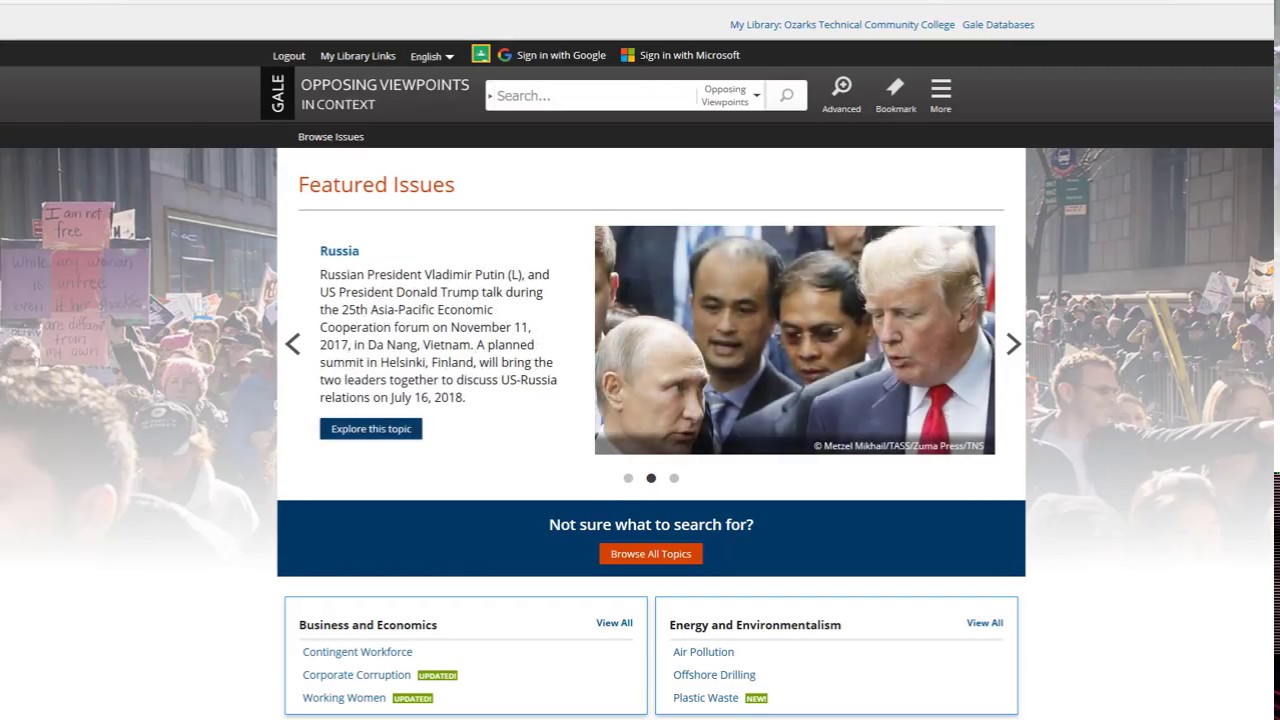The top section of the website is dominated by a gray banner featuring small blue text, which appears to include the phrase "My Library." The exact additional wording is unclear due to the text size. Beneath this, there is a black and gray navigation bar offering options such as "Logout," "My Library," and "English." This bar also hosts several icons: a green square icon, the Google icon accompanied by "Sign in with Google," and the Microsoft logo next to "Sign in with Microsoft."

The main content area starts with the title "Opposing Viewpoints in Context" prominently displayed to the left near the G-A-L-E logo. Adjacent to it on the right is a white search field flanked by three clickable white icons, with the last one identified as a menu.

A notable section titled "Featured Issues" is highlighted within a white box featuring red text. At the center, there is a photograph displaying Russian President Vladimir Putin and U.S. President Donald Trump engaging during the 26th Asia-Pacific Economic Cooperation Forum. Brief descriptive text accompanies the image. Below this photograph, a blue button offers additional engagement.

Further down, a blue banner prompts users who might be uncertain about what to search for, accompanied by an orange clickable button. At the bottom of the page, there are two distinct square sections focusing on different areas: one dedicated to "Business and Economics" and the other to "Energy and Environmentalism."